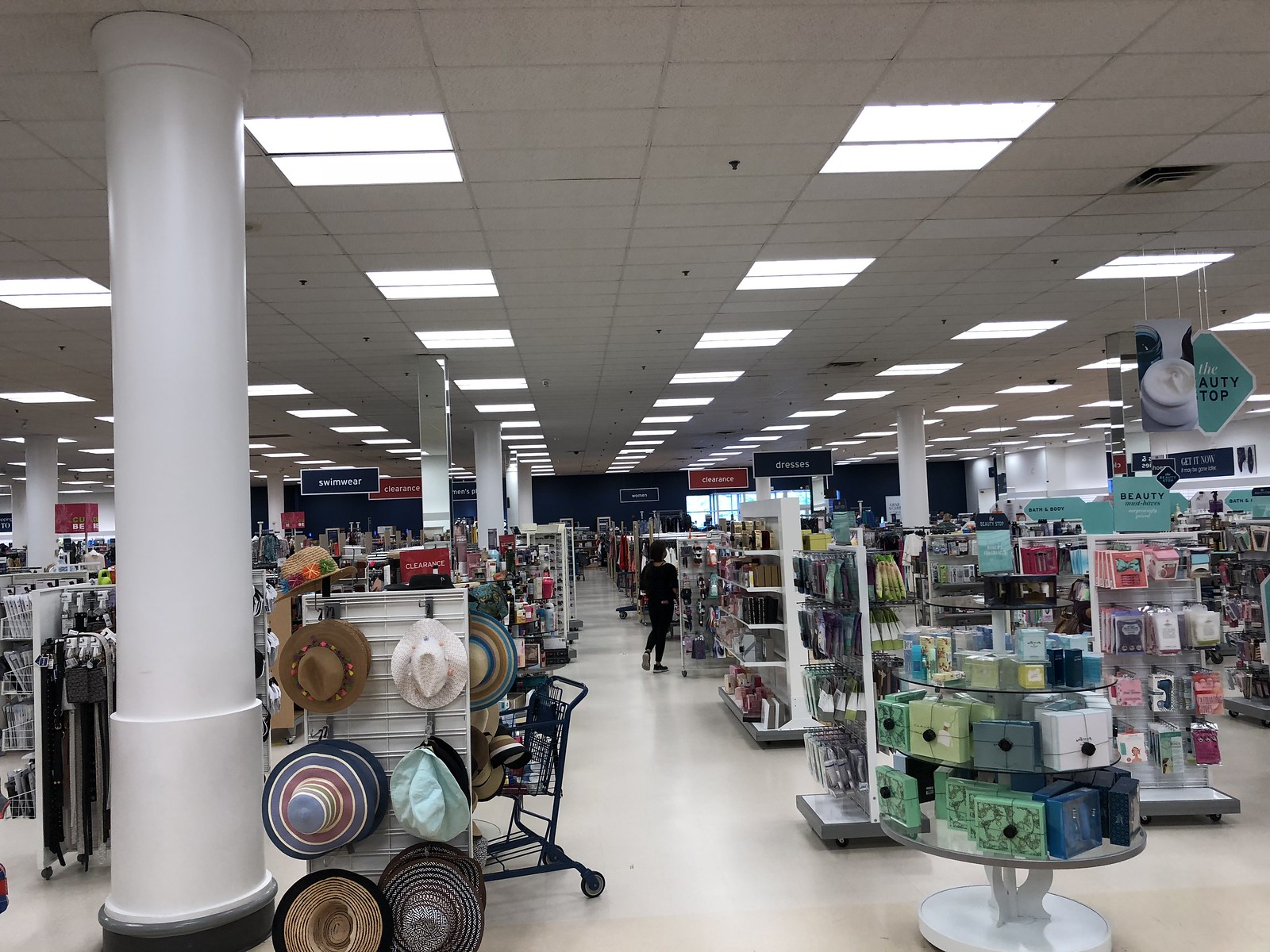The photograph captures the interior of a store, showcasing a clean and organized environment under a white, drop-style ceiling. The ceiling is illuminated by fluorescent lighting, which provides a bright, even light throughout the space. To the left of the image, a prominent white column extends from the ceiling down to the floor, adding to the structural aesthetic of the store.

Next to this column stands a white hat rack adorned with an array of colorful hats. From top to bottom, there is a tan hat embellished with brown and orange decorative pieces, followed by a white hat. Below these, a vibrant hat displaying blue, red, and gold stripes catches the eye. Adjacent to this is a mint green hat, and beneath the striped hat sits another tan hat featuring a black brim. Completing the collection, a gray hat is positioned next to the second tan hat.

A shopping cart is visible behind the hat rack, hinting at the bustling activity within the store. To the right side of the image, shelves stocked with an assortment of colorful boxes—green, blue, white, and gray—add a lively touch to the scene. In the background, various beauty products are arranged along numerous aisles, each filled with a wide array of items.

The overall scene portrays a well-stocked store with diverse merchandise displayed in a neat, orderly manner, offering customers a pleasant shopping experience.